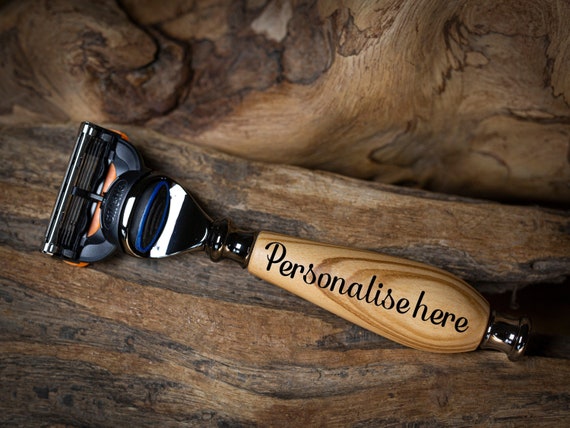The image showcases a sleek, contemporary razor with a sterling silver or silver knob, resting on a natural, multicolored wooden surface. The razor features a modern design, with a sophisticated head and connection. The handle is crafted from light-colored wood, adorned with elegant wood rings and marked with the words "personalized here," suggesting customization options for personal use or business purposes. The wooden background enhances the natural aesthetic of the scene, showing unstained, authentic wood grains and knots. The razor itself bears traces of orange, black, and blue near the head, and although a brand name is present in black, it blends into the handle, making it difficult to discern.